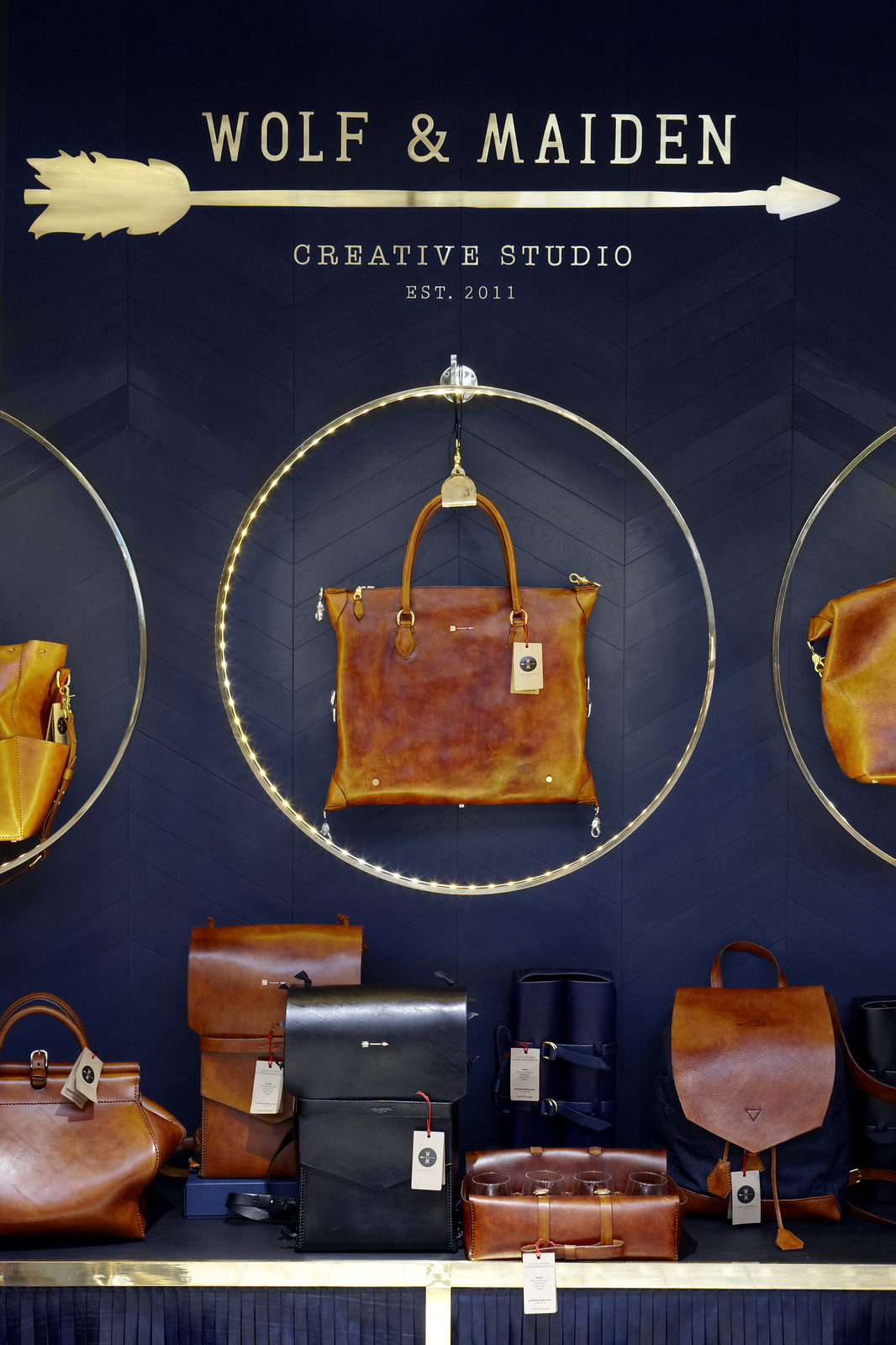This is a vertical rectangular advertisement for "Wolf and Maiden." The background transitions from black at the top to dark navy at the bottom. At the very top left, the shop's name, "Wolf and Maiden," is written in reflective gold letters that fade lighter across, accompanied by a rightward-pointing gold arrow. Beneath the name is the tagline, "Creative Studio," and "Established 2011" in white letters.

The image prominently features several leather bags and accessories. The center highlights three gold circles hanging from hooks, with the central circle fully visible, displaying a brown leather bag adorned with multiple zippers and a tag. The circles on either side are partially cropped, showing portions of other leather bags.

Below the circles, a silver shelf holds additional leather goods, including a brown handbag with two handles, a brown and a black backpack, and another satchel bag, all tagged. The photographic style merges representational realism with graphic design and typography.